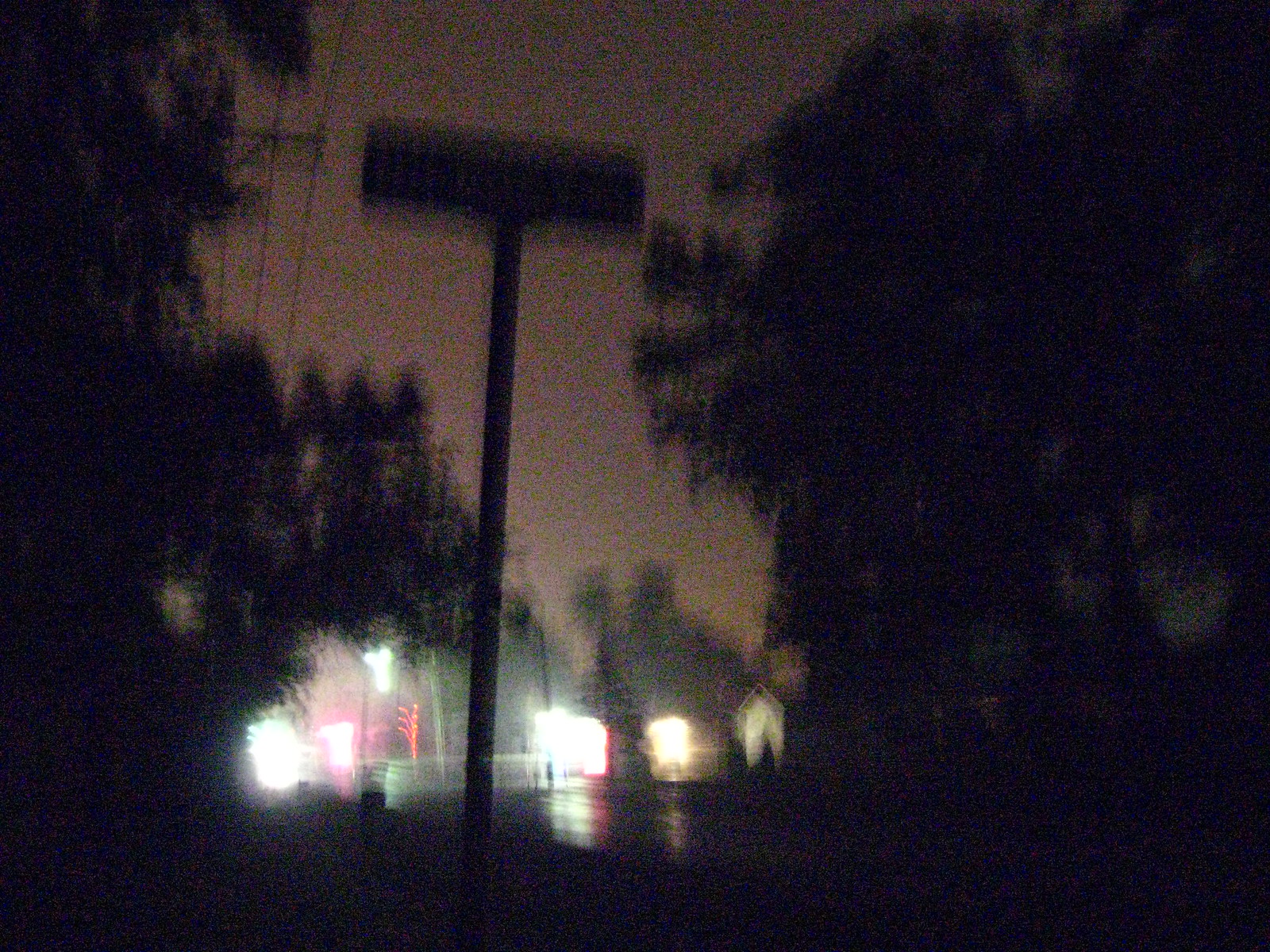This image captures a blurry, nighttime scene likely taken in motion, obscuring precise details. The setting appears to be a residential street or a roadway bordered by trees, evident on both the left and right sides of the picture. These trees suggest the area might be on the edge of or emerging from a forested region. Power lines can be faintly seen above the trees on the left side. The sky above is a murky brownish-purple hue, transitioning to a pinkish-red at the top center. In the middle-ground, there is a small structure that resembles a shed, surrounded by indistinct, glowing lights creating a distorted, streak-like effect. A cylindrical pole with a rectangular, possibly road or street sign is visible off-center to the left, though the sign's text is unreadable. Overall, a strip of reflective black, likely the street, runs through the center, amplifying the blurred lights and adding to the image's sense of movement and low visibility.